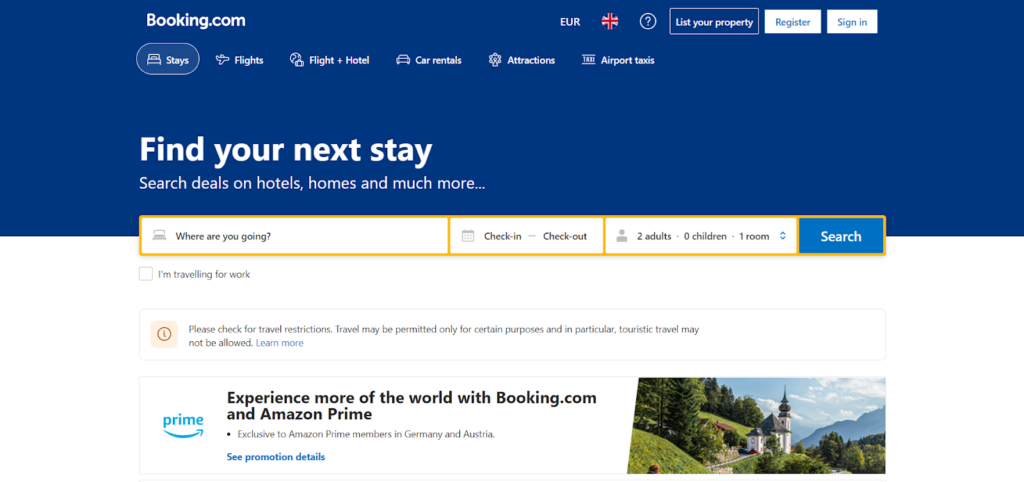The image depicts a webpage from the well-known travel website Booking.com. The upper half of the page is characterized by a blue background, while the lower half features a white background. Prominently displayed in white text on the top left is the Booking.com logo.

Below the logo, there are several navigation tabs, each for a different type of booking service: "Stays," "Flights," "Flight + Hotel," "Car Rentals," "Attractions," and "Airport Taxis." The "Stays" tab is highlighted.

In the upper right corner, there are several options including a currency setting displaying "EUR" alongside the UK and EU flags, a "Help" link, and a "List Your Property" link. Additionally, there are buttons for "Register" and "Sign In," both displaying white text on a blue background.

In the center of the page, dividing the blue and white sections, is a search box with a yellow border. It features fields for entering travel details: "Where are you going?" "Check-in" and "Check-out" dates, "2 adults," "0 children," and "1 room." To the right of these fields is a blue "Search" button. Below this, there is a checkbox labeled "I am travelling for work." 

A travel advisory is displayed beneath the search box, cautioning users to check for travel restrictions as travel may be limited to certain purposes with tourist travel potentially disallowed. A prompt encourages users to "Learn More" for additional details.

At the bottom of the page is a promotional section linking Booking.com services with Amazon Prime. It reads, "Experience more of the world with Booking.com and Amazon.Prime. Exclusive to Amazon Prime Members in Germany and Austria, see promotion details," accompanied by a blue call-to-action button.

On the right side of the page, a picturesque image features a verdant landscape with green trees, rolling mountains, and a blue sky. In the foreground, there is a building with white walls and a grey roof, complementing the serene nature scene.